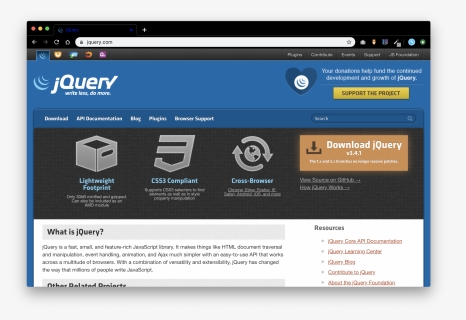Caption: 
A nostalgic screenshot captured from an early web page dedicated to jQuery, a popular JavaScript library designed to simplify HTML document traversing, event handling, and animation. The minimalist and somewhat dated design indicates its origin from an earlier era of web development. Prominently displayed are three key benefits of jQuery: a lightweight footprint, CSS3 compliance, and cross-browser compatibility. A noticeable "Download" button implies the availability of the software for immediate use, with "jQuery.exe" appearing in the search menu, suggesting the user was specifically looking for an executable file of this software. The text is quite small, making it difficult to read, but the overall purpose of the page—to facilitate jQuery downloads and highlight its advantages—is clear.